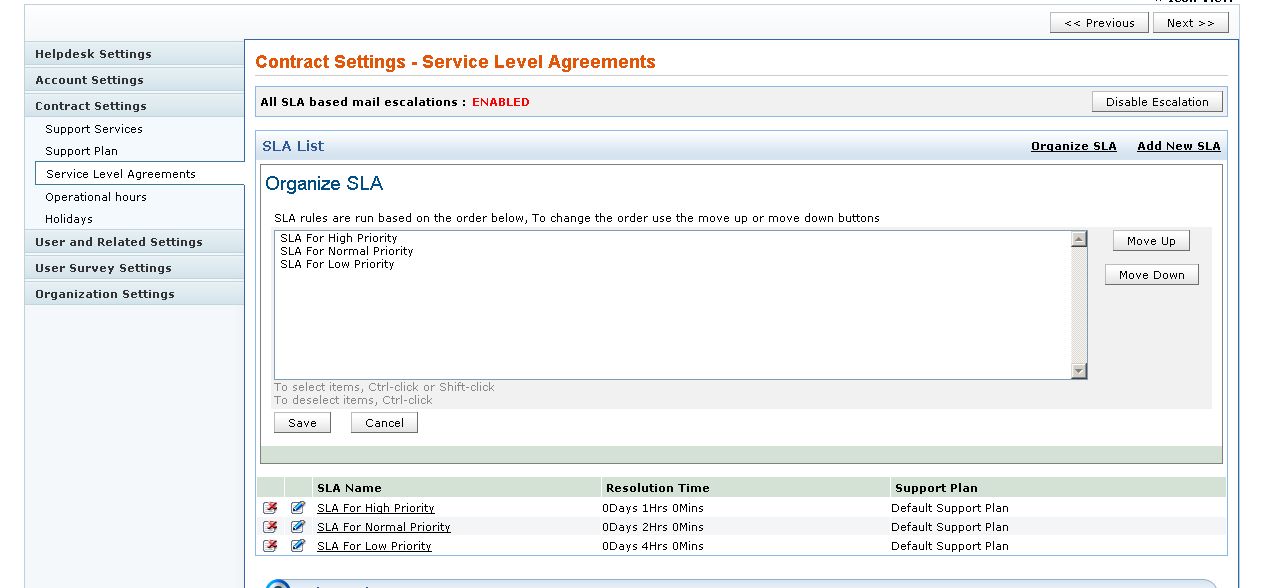This image showcases a detailed view of someone's help desk settings area, specifically under the "Contract Settings" section. The user has navigated to and clicked on the "Service Level Agreements" option. At the top of the screen, in orange text, it reads "Contract Settings" followed by "Service Level Agreements."

Further down, there's a prominently highlighted section labeled "All SLA Based Mail Escalation" with "ENABLED" displayed in bold, red, uppercase letters. Below this, a section titled "SLA List" is visible, which includes a button labeled "Organize SLA."

The following text explains that "SLA rules are run based on the order below. To change the order, use the move up or move down buttons." The list beneath details different SLAs (Service Level Agreements) for various priority levels: high, normal, and low, each accompanied by arrows allowing the user to reorder them as necessary.

At the bottom of the screen, there's a note explaining how to select items ("control click" or "shift click") and how to deselect items ("click, click"). Finally, there are buttons for saving or canceling any changes made to the settings.